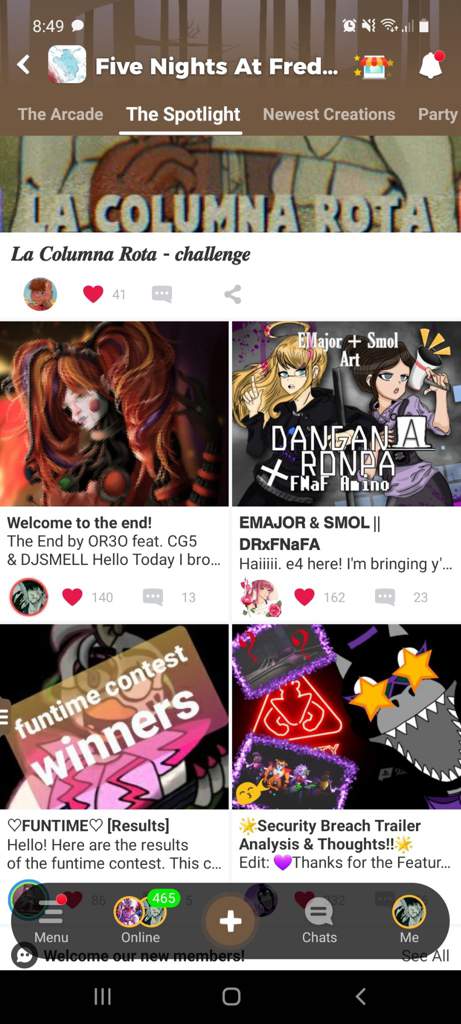This screenshot showcases an Android application interface, seemingly related to the "Five Nights at Freddy's" franchise, as indicated by the title visible at the top. The UI includes a notification icon represented by a bell with a dot. Centrally featured is a section titled "La Columna Rota Challenge," which appears to be a Spanish title and suggests a video-watching challenge or event.

Below this section are four distinct categories related to "Five Nights at Freddy's." The top two categories each feature female characters and seem to be fan art. The bottom left category is labeled "Funtime Contest Winners" and likely highlights winners of a user-submitted content contest. The bottom right category is titled "Security Breach Trailer Analysis and Thoughts," suggesting a reaction or analysis video of a game trailer.

Navigating further down, the application’s user interface displays several function buttons. From left to right, these include:
1. **Menu** - for navigating various app sections.
2. **Online** - presumably indicating the number of active users.
3. **Plus Sign (+) in a Circle** - possibly for creating new posts or content.
4. **Chats** - for accessing message communications.
5. **Me** - likely leading to the user's profile page.

Overall, the screenshot provides a detailed look at an app devoted to "Five Nights at Freddy's" with fan art, contests, video analyses, and a robust user interaction framework.